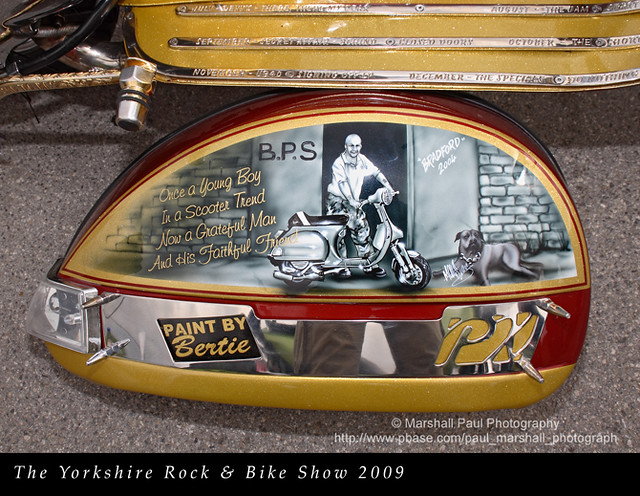This advertisement for the Yorkshire Rock and Bike Show 2009 features a detailed and nostalgic image. The focal point is what appears to be a wheel well or side cap from an old-fashioned scooter, resting on a surface that resembles either concrete or tile. The artwork painted by Bardi (or Bertie) portrays a black and white scene of a man standing beside his scooter with a dog sitting faithfully by his side. The background reveals a brick-lined alley with a warehouse-like door marked partially with "BPS". Emblazoned in gold-yellow lettering, the caption reads, "Once a young boy in a scooter trend, now a grateful man and his faithful friend." The artwork is accentuated with chrome and red trim. Additionally, the bottom part of the image includes text in white that announces "The Yorkshire Rock and Bike Show 2009". The artist's credit, "Paint by Bardi," along with photographic credit to "Marshall Paul Photography" and a URL, are also present, giving the piece a rich and storied visual that captures both the spirit of the event and the passage of time.